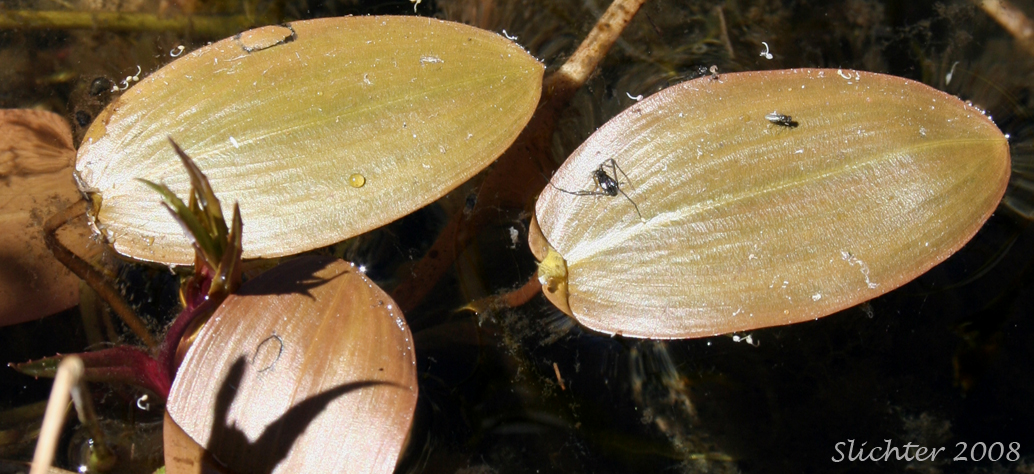The image showcases three leaves floating on water, exhibiting various shades of vibrant green and earthy brown tones. The leaves are arranged with one in the upper left, one in the middle right, and another towards the bottom left. The leaf in the upper left has a small water droplet towards the bottom and a stem connecting it to another leaf below. A shadow of a stem is visible on this leaf due to a light source outside the frame. The leaf in the middle right hosts two small black insects, one positioned toward the left and another near the upper right. The background remains largely indistinct due to blurriness, emphasizing the leaves and their details. In the bottom right corner, the image is watermarked with "Slichter 2008."